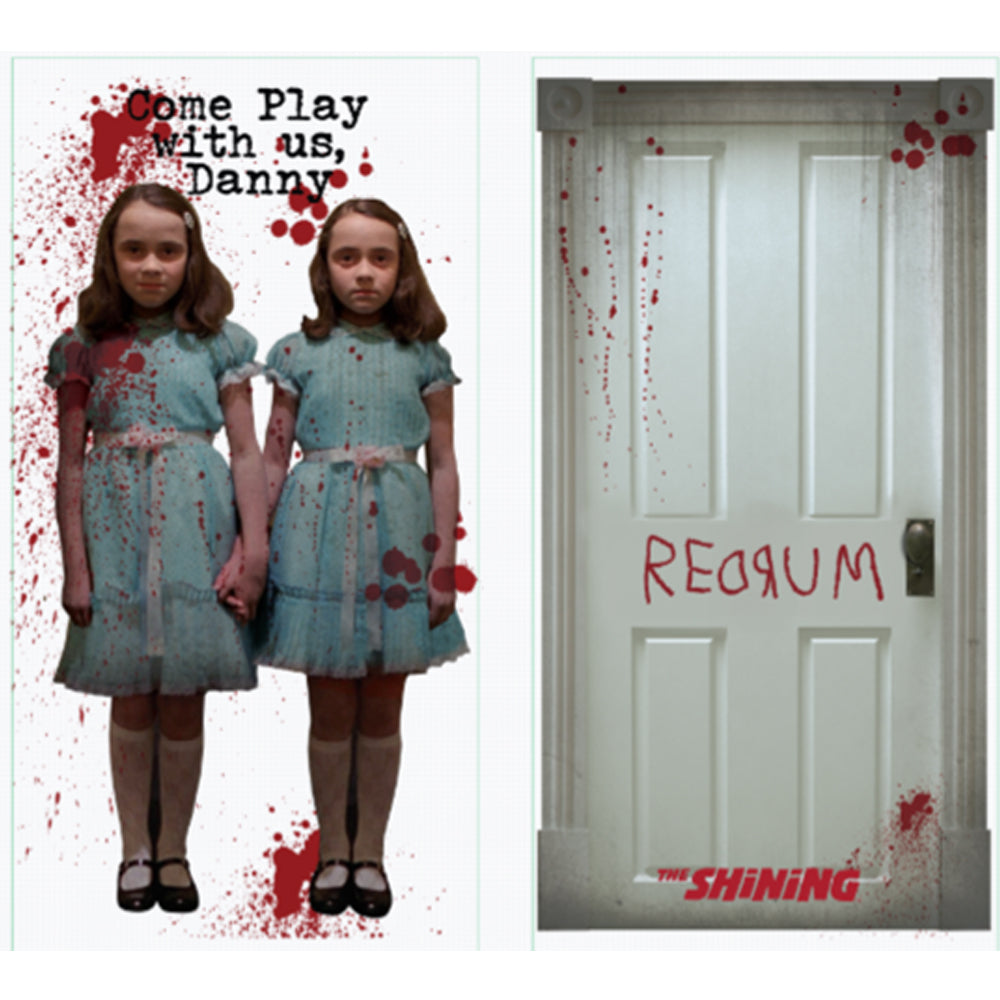The scene from the movie *The Shining* features two twin girls on the left side, each with long brown hair and a haunting stare. They are dressed identically in light blue dresses with white belts, lace trim at knee level, long white socks, and black leather shoes with straps. Above the girls, the text "Come play with us, Danny" is displayed in black. Bloodstains are splattered on the girls, their dresses, the floor, and the wall behind them. On the right side, there is a white door with bloodstains concentrated on the bottom right, top left, and top right. The word "REDRUM," spelled backwards with the letters "T" and "R" written in reverse, is prominently written in red at the center of the door. The bottom of the door features the movie's title, "The Shining," also written in red. The doorknob is positioned on the right side of the door.